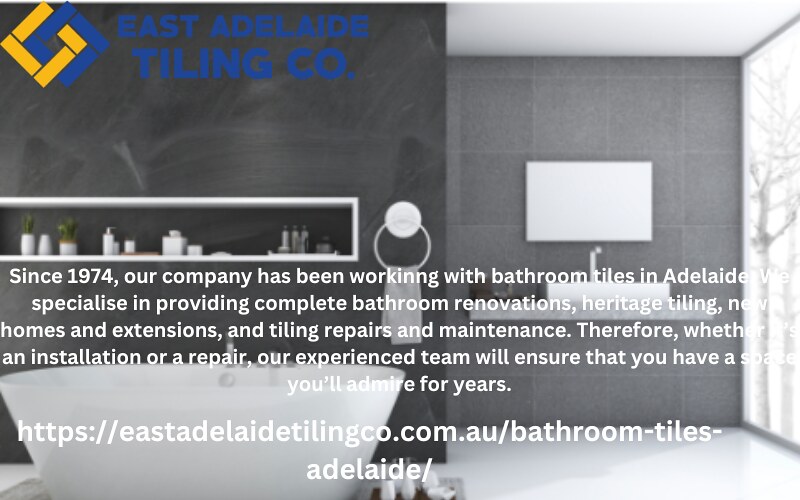The image is an advertisement for East Adelaide Tiling Company, featuring their logo composed of two overlapping diamond shapes—one gold and one royal blue. The company name, "East Adelaide Tiling Company," is prominently displayed in royal blue font. The ad's backdrop includes a grayish-black, tile-like texture with elements such as a sketch of some trees and a lamp in the background. The main text, in white font, states: "Since 1974, our company has been working with bathroom tiles in Adelaide, specializing in complete bathroom renovations, heritage tiling, homes and extensions, and tiling repairs and maintenance. Whether it's an installation or repair, our experienced team will ensure that you have a space you'll admire for years." The company's website links are http://eastadelaidetilingco.com.au and bathroom-tiles-adelaide.com. The image appears somewhat fuzzy and unclear, and there are elements like a bathtub, sink, and towel rack visible in the background.